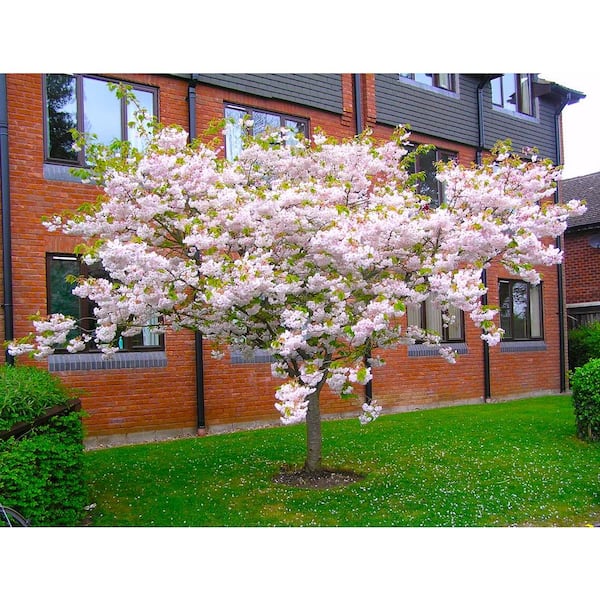This outdoor image features a picturesque scene dominated by a small tree adorned with an abundance of pink and purple blossoms, interspersed with green leaves. The tree, standing approximately eight to ten feet high, boasts a profusion of blooms starting about two feet from the ground and continuing upward, creating a cascading effect of vibrant flowers. The branches spread asymmetrically, giving the tree a charming, floofy appearance. Beneath the tree, the well-kept green grass is scattered with fallen petals, adding to the scene's natural beauty. Surrounding the tree are various bushes and hedges, with some located towards the lower left and others towards the middle right of the image.

In the background stands a three-story red brick apartment building, characterized by black borders under the windows and sections of dark gray or black siding near the top floor. The building features numerous windows and some visible black gutters. Partially visible to the upper right is a bit of the sky, appearing white. The setting is further enhanced by glimpses of another similar building on the right-hand side, contributing to the overall impression of a serene residential area in full bloom.